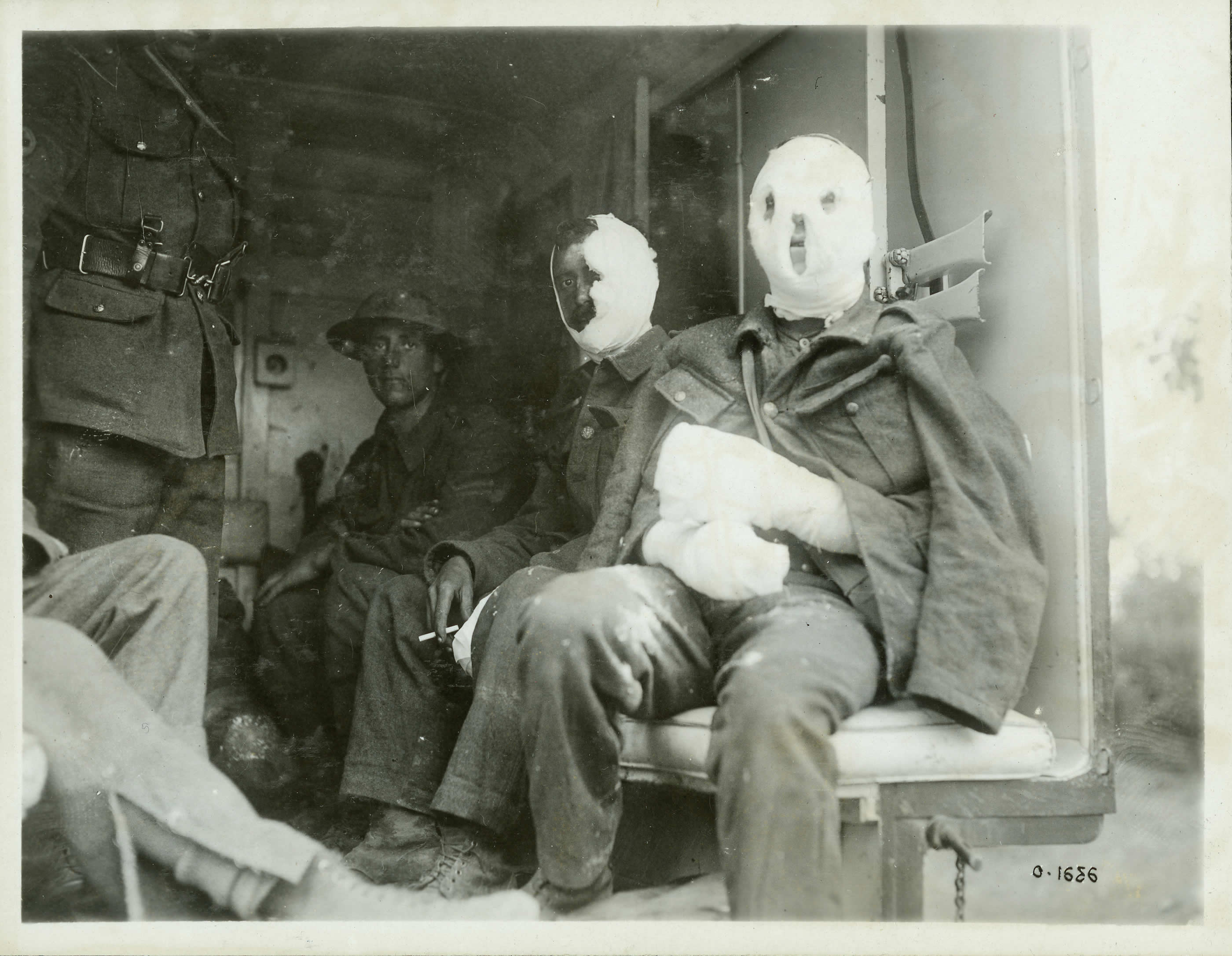This is a detailed black-and-white photograph from an old military scene, capturing a group of men in the back of a truck or medical ambulance. In the center, a man dressed in full army gear, including a hat, sits next to another soldier with bandages covering half his face and boots on his feet. Further to their left is a man heavily swathed in gauze, covering his entire face and hands, suggesting injuries, and he is also clad in a coat, pants, and boots. Another individual, partly visible, sits to the far left, wearing jeans and boots. Adjacent to them, there’s a person in a military uniform distinguished by a black belt with silver buttons and black pants, appearing to look outside the vehicle. The interior of the van is white, with the dirt visible on the floor and some in the background. The image, marked with the number 0-1636 at the bottom right, shows these men seated on the side benches typically found in such military transport vehicles.